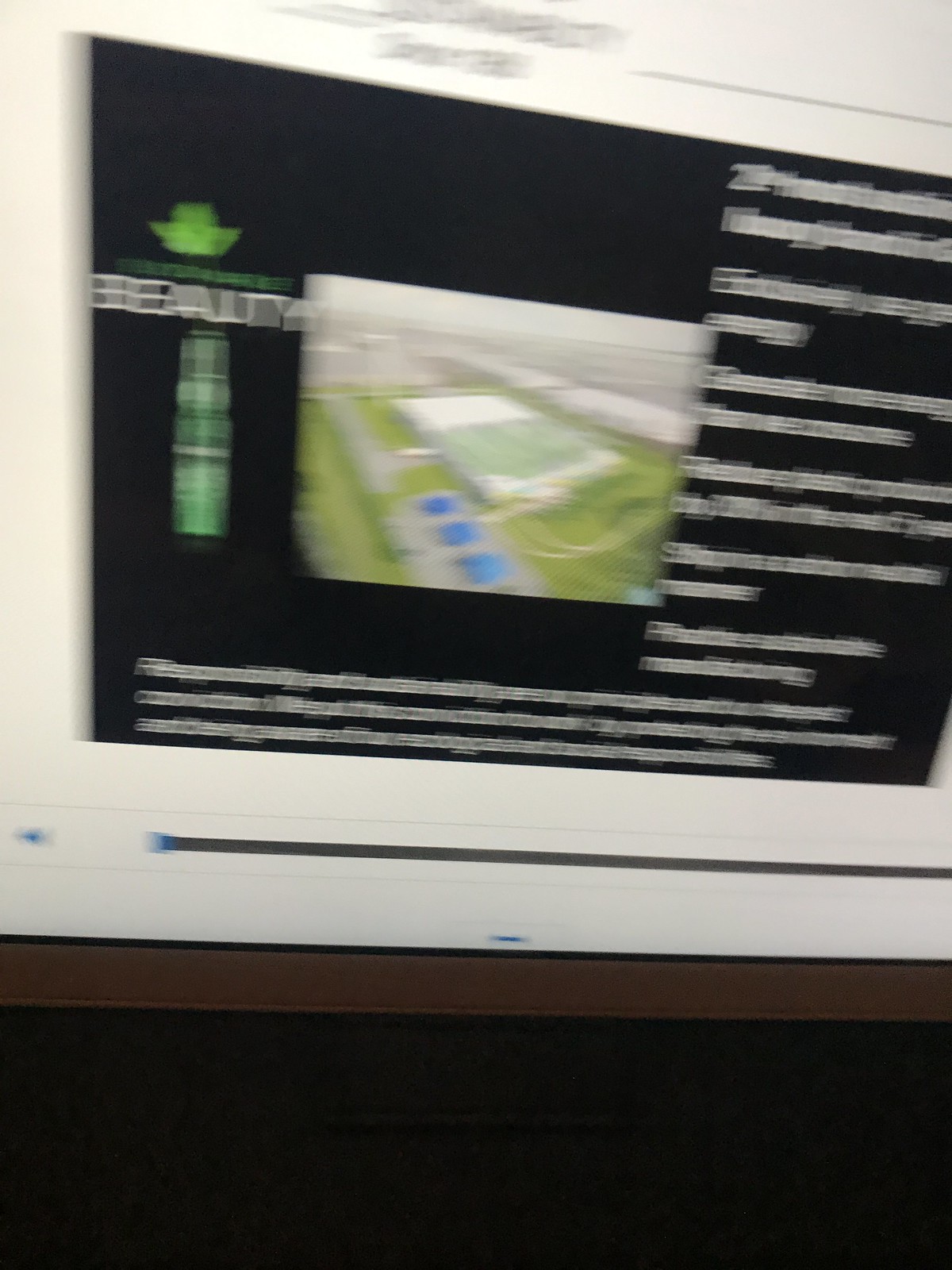This image is a vertically rectangular photograph capturing the display of a computer monitor. The photograph is notably blurry, making the details less discernible. The monitor's overall background is white, while the central area of the screen features a black backdrop with white text. At the core of this black background, there is an aerial image, although its clarity is compromised by the blurriness. On the right side of the aerial image, white text is visible, but the specific details of the verbiage are obscured. 

The monitor also features a white border area around the display. On the left-hand side of this border, a small blue icon is present. Adjacent to it, stretching horizontally to the right, is a long black slider with a blue dot positioned on the left end of the slide. This setup suggests the presence of a video player or a similar interface, though the blurriness of the photograph prevents a precise identification.